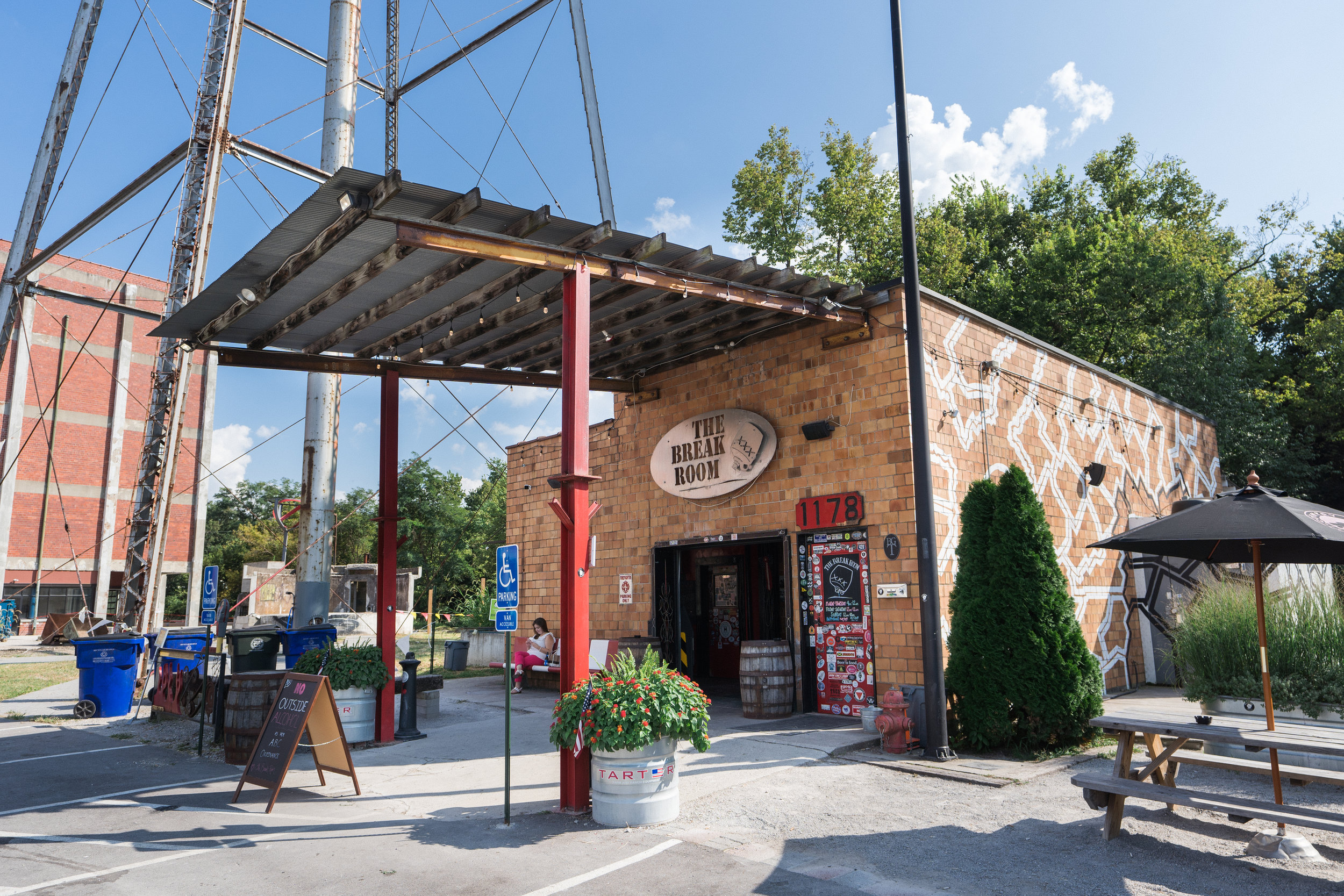In this detailed daytime photograph taken under a sunny sky with a few white clouds, we see a coffee shop named "The Break Room," prominently featuring a white oval sign with the store name and an image of a coffee cup pouring out coffee. The central structure of the scene is a red brick building at address 1178, adorned with a red door decorated with stickers and a large bay door. The entrance is highlighted by a sign above that reads "The Break Room" in silver.

To the right side of the building’s entrance, there is a cedar tree. Adorning the area is a can repurposed as a flower pot, filled with vibrant red flowers and green leaves. A picnic table with a black umbrella provides a cozy outdoor seating area. The structure includes a canopy similar to that of a gas station, supported by two steel posts and attached to the building, creating a sheltered area for visitors.

Amidst the scene, we observe a blue handicap parking sign adjacent to a designated parking bay, with other parking spaces visible. Adding to the charm, a chalkboard sign stands in front, although the writing on it is not legible. The surrounding area features four blue rubbish and recycling bins and a tall red brick building in the background. Enhancing the picturesque setting are very tall green trees and a large telephone tower situated behind the bins and the shop.